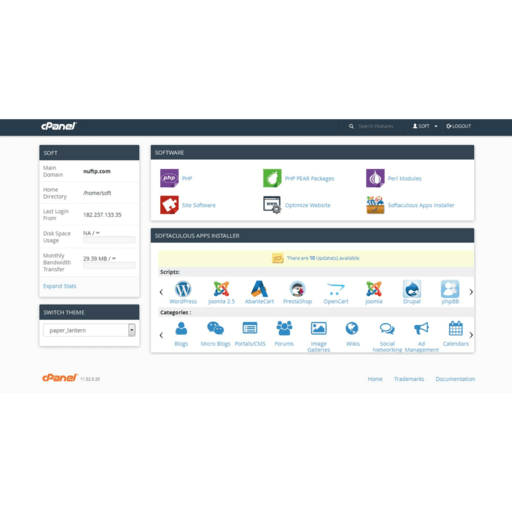A screenshot of a web hosting dashboard interface reveals an organized layout designed for efficient management. At the very top, a dark grey bar spans across the width of the screen, prominently displaying "cPanel" in clean, white text on the left-hand side. Directly beneath this bar, a vertical sidebar is anchored on the left, divided into two distinct sections. 

On the main area to the right of the sidebar, two larger sections dominate the view, each section demarcated by its own dark grey bar running horizontally at the top. In addition to mirroring the header bar's color, these smaller bars help to visually segment the content below them. The overall aesthetic is consistent, featuring a modern and professional design.

Toward the bottom left corner, the word "cPanel" appears again, this time in a vibrant orange, adding a splash of color to an otherwise subdued palette and reaffirming the platform's branding. This detailed layout ensures that users can navigate the dashboard with ease, leveraging the clear structure for optimal functionality.